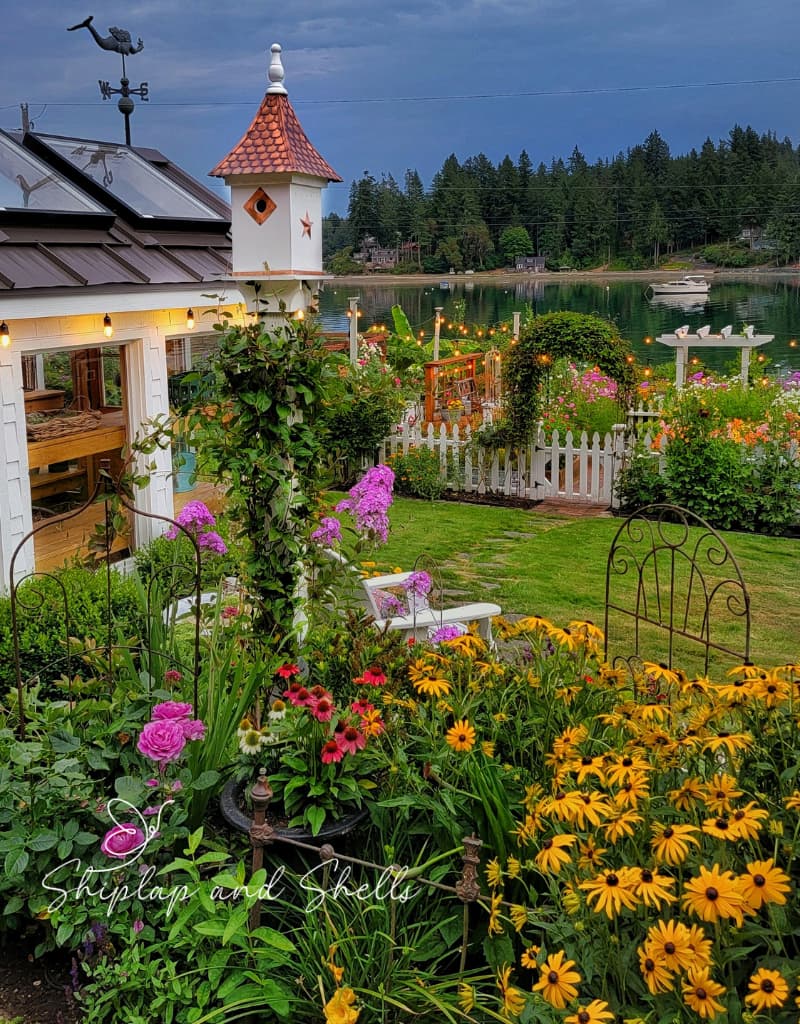This photograph captures a picturesque flower garden situated outside a pristine white home with a brown roof. The meticulously manicured green lawn stretches across the scene, bordered by a charming white picket fence. The garden is a kaleidoscope of colors with an abundance of flowers including lilies, carnations, roses, black-eyed Susans, and various pink, yellow, purple, and red blooms. Vines climb up trellises, posts, and an iron gate, adding to the lush texture of the garden. 

In the center of this floral paradise sits a white lawn chair, invitingly set amidst the vibrant blossoms. The yard features a small walkway leading to the white picket fence, beyond which lies a tranquil lake. A small boat floats on the lake's surface, framed by a cluster of hardy green cedar trees on the opposite shore. The backdrop is completed by a blue sky stretching into the distance. 

The home behind the garden boasts a brown roof, large moon roofs, French doors that open to reveal wood floors inside, and a patio with a weather vane on top. The patio features white posts adorned with lights, and from its edge, the garden spills forward in a riot of color. An iron gate and a pergola arch adorned with climbing vines further enhance the garden's charm. 

Overlaying this idyllic scene is text that reads "Shiplap and Shells," adding a quaint touch to the overall composition.